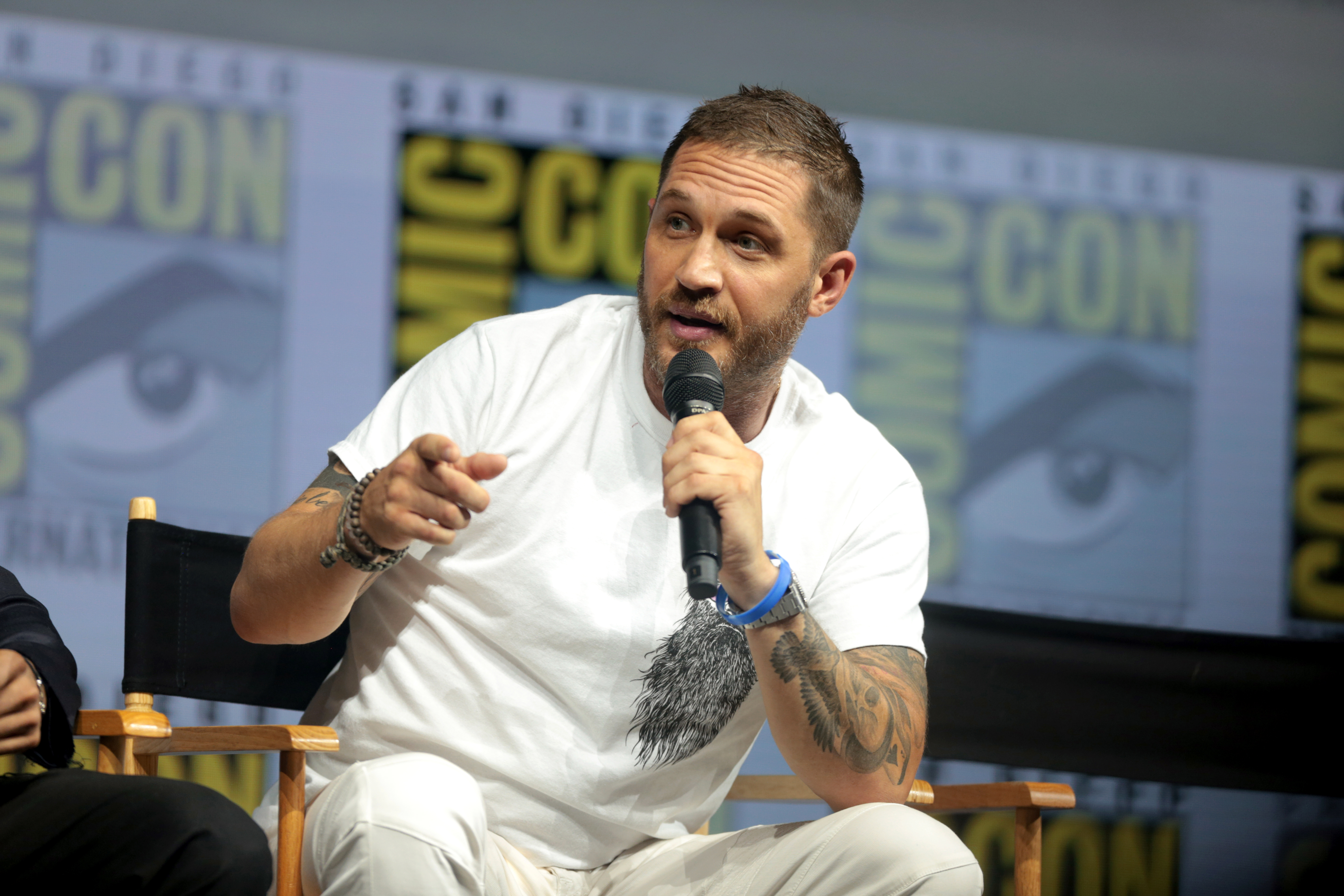In the image, a man is seated on stage at Comic-Con, indicated by a backdrop displaying the Comic-Con logo in black and yellow lettering, and partly obscured posters featuring an eyeball. He sits in a black director-style chair with wooden arms, leaning forward with one elbow resting on his knee, as he speaks into a microphone held in his tattooed left hand. His tattoos include a skull and a bird. The man, who has styled short hair, a mustache, and a closely shaped beard, is dressed in a white t-shirt with a black design on the left breast and white pants. His expressive face shows lifted eyebrows and forehead wrinkles. He points toward someone off-camera with his right hand, while another person sits beside him. Accessories such as bracelets and a watch adorn his wrist, adding to his detailed appearance.